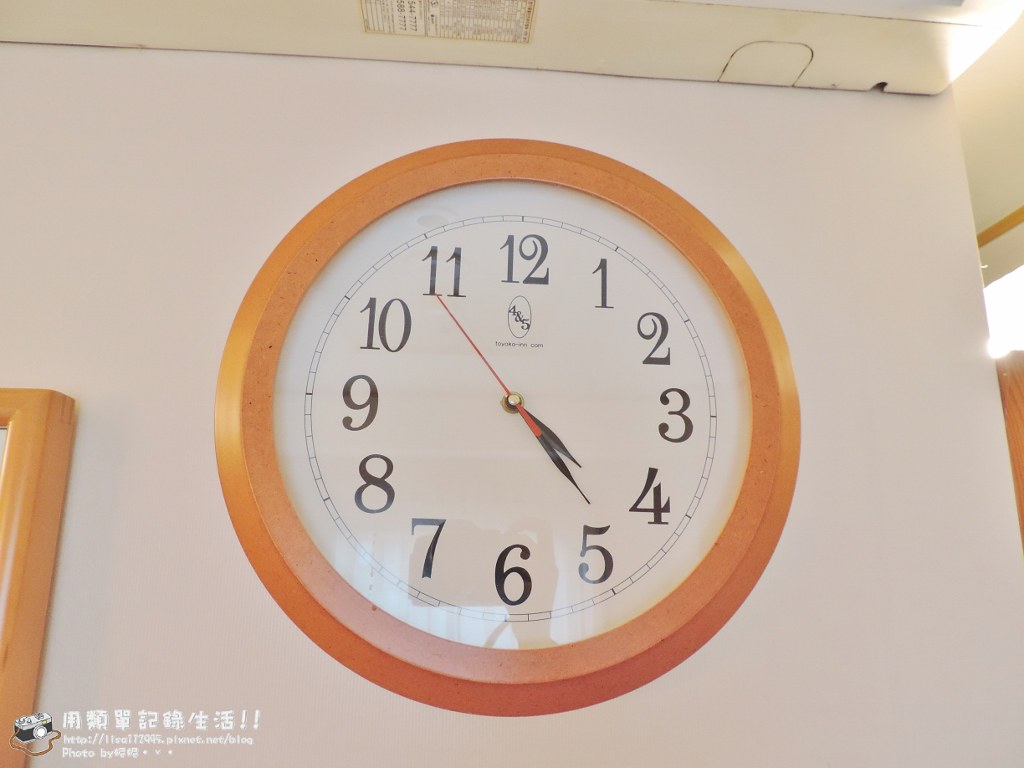The image features a wall-mounted clock with an elegant light brown wooden frame. The clock face displays the numerals 1 through 12 in a clear, easy-to-read font. A small, indistinct logo or name is present near the center, though it is not easily legible. The clock has two black hour and minute hands, along with a red second hand, indicating the current time as 4:24. In the lower left corner of the image, there is some non-English text. Additionally, the image includes a camera with a neck strap, positioned against the wall, adding an element of interest to the scene.